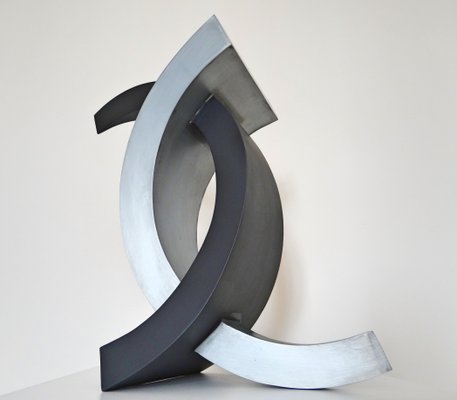The photograph features a modern sculpture set against a pristine white background, possibly displayed in a museum. The artwork depicts two intertwined, crescent-like arcs that merge to create a single, cohesive piece. Each arc resembles approximately 40% of a circle and together they form a diamond-like shape where they intersect. One arc is a sleek silver, oriented to the right, while the other is a bold black, facing left. These half-moon shaped steel pieces appear as though they are entwined or seemingly glued together, symbolizing unity and togetherness despite differences. The juxtaposition of the silver and black elements serves to convey a deeper message of harmony between contrasting entities.